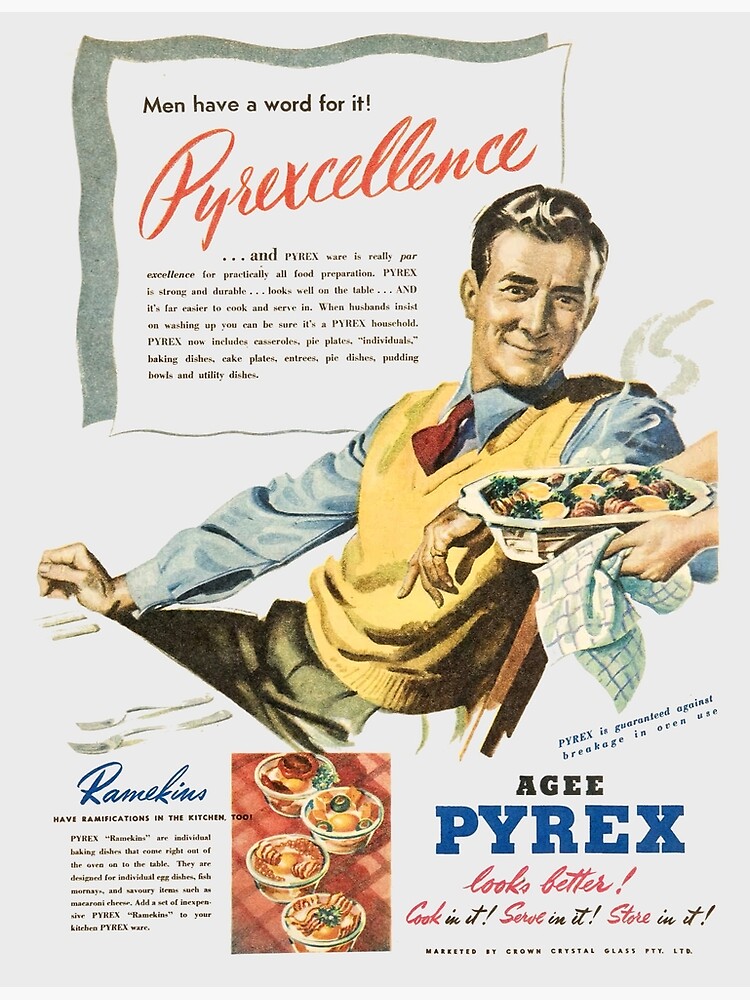This vibrant, vintage advertisement from the mid-20th century, likely the 1940s or 1950s, showcases the superior quality of AGEE Pyrex cookware. Dominating the white background is a colorful illustration of a jovial, middle-aged man with short, dark hair, dressed in a yellow sweater vest over a blue long-sleeve shirt and a red tie, and greenish pants. Seated at a table set with a knife, fork, and a welcoming ambiance, he eagerly gazes to his right at a steaming hot casserole dish being presented to him. The dish, held by unseen hands using protective towels, emanates warmth and deliciousness, hinting at its superb preparation in Pyrex cookware.

Above the illustration, a bold red cursive tagline proclaims, “Men have a word for it, Pyrexilence,” emphasizing the cookware’s excellence. Below, descriptive text praises Pyrex for its strength, durability, and aesthetic appeal, affirming it as the go-to choice for cooking, serving, and storing food. Additional text highlights the extensive range of Pyrex products, including casseroles, pie plates, baking dishes, and utility dishes, all guaranteed against breakage and suitable for oven use.

On the bottom left, images of various Pyrex dishes filled with enticing food further illustrate the cookware's versatility and appeal, while the bottom right corner proudly states, “AGEE Pyrex looks better cooking it, serving it, storing it,” marketed by Crown Crystal Glass Pty. Ltd. This nostalgic ad elegantly combines the cheerful anticipation of mealtime with the unmatched quality and reliability of Pyrex cookware.